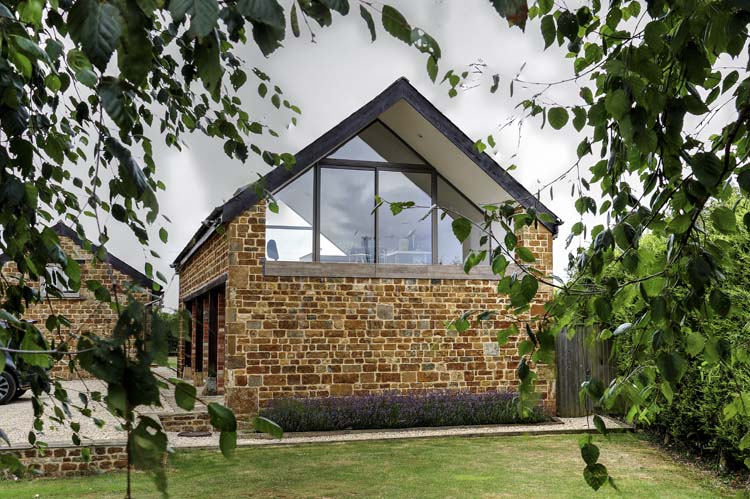The photograph, taken in landscape orientation, captures an outdoor scene featuring a well-maintained estate. Dominating the image are two adjacent brick buildings with distinctive dark V-shaped roofs. The primary structure, likely a main house, features clear windows with brown sills. To its left, partially visible behind greenery, is a secondary building that appears to be a garage or an outhouse.

The top corners of the photo are framed by overhanging green leaves, suggesting the picture was taken from behind a tree. Below, the neatly mowed lawn is complemented by a gravel walkway that leads to a driveway, where a partial view of a car is visible in the lower left corner. The lower right corner shows additional bushes and greenery, contributing to the lush, well-kept appearance of the estate.